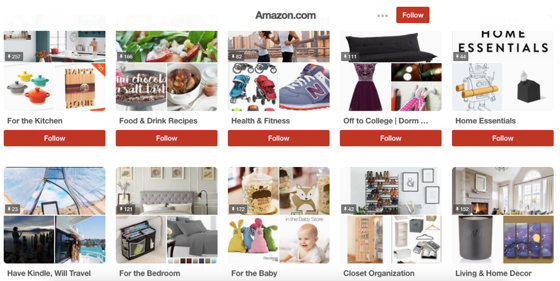This image depicts an Amazon list option, strikingly reminiscent of Pinterest boards, aimed at various aspects of daily life. Prominently, the Amazon logo, along with "amazon.com," is positioned at the top center. The screen features several categorized boards, each dedicated to specific interests and necessities.

1. **Home and Kitchen:** This board showcases a diverse collection of items, prominently featuring four crock pots in different hues—yellow, teal, gray, and red. A sign reading "Happy Home" is displayed alongside a modern kitchen photograph accented in blue and white tones.
2. **Food and Drink Recipes:** A variety of recipes are displayed, including a depiction of a French dip sandwich accompanied by an au jus on the bottom right.
3. **Health and Fitness:** This section includes images of a Nike shoe, jogging strollers, and two individuals engaged in a run.
4. **Off to College Dorm:** Essential dorm items such as a futon, a dress, and various hanging supplies are highlighted here.
5. **Home Essentials:** This board offers an array of intriguing Amazon finds tailored to diverse needs, featuring items like a robot that has two hooks, possibly serving as a closet organizer.
6. **Have Kindle, Will Travel:** A captivating collection of travel photos is presented on this board.
7. **For the Bedroom:** This section showcases a gray tufted headboard alongside some linen sheets.
8. **For the Baby:** It highlights numerous baby toys and a charming photograph of an infant.
9. **Closet Organization:** This board provides numerous ideas for organizing closets efficiently.
10. **Living and Home Decor:** Depictions include various photos, a candle, and an illustration of a beautifully designed modern living room. 

The comprehensive nature of the boards exemplifies the versatility and breadth of the products and ideas available on Amazon, making it a go-to resource for a multitude of lifestyle needs.